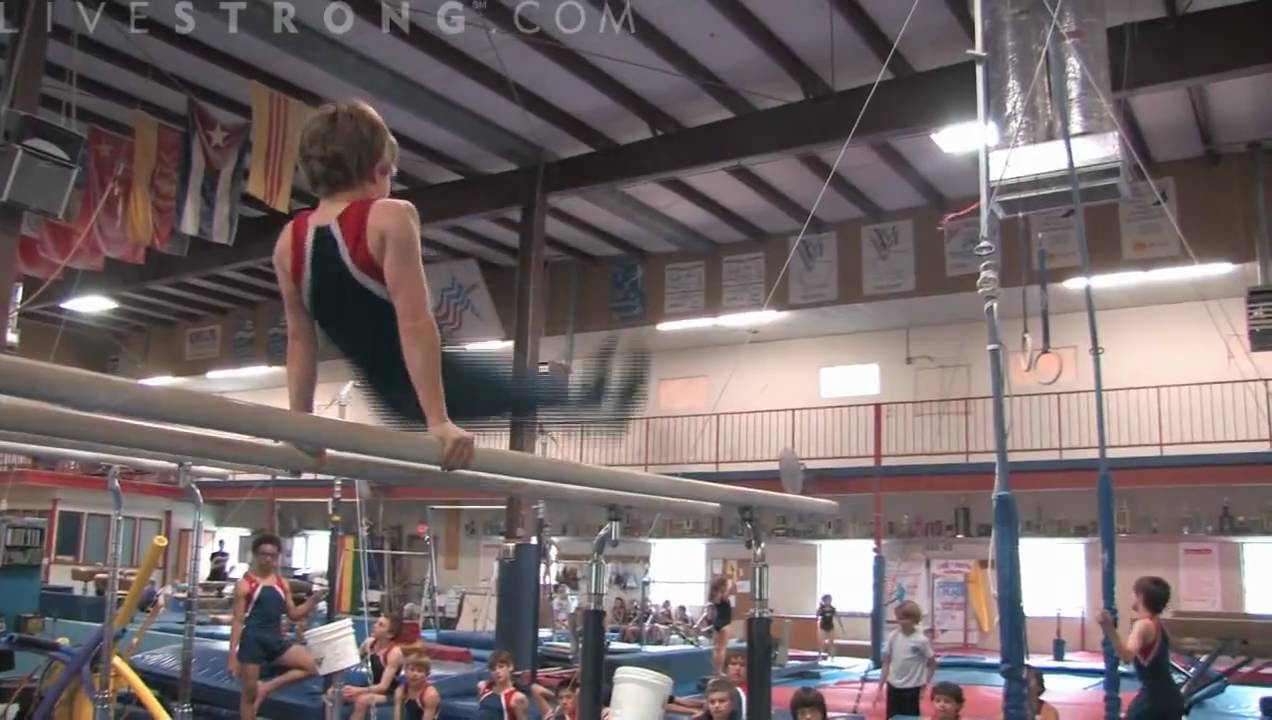The photograph captures a vibrant scene inside a gymnasium adorned with metal beams and a second-floor walking track with railings. Prominently featured in the foreground to the left is a young male gymnasts of Caucasian descent, clad in a black and red unitard, performing an exercise on parallel bars. His hands are gripping the light brown bars firmly, lifting his body with legs extended out, indicating dynamic motion. Beneath him, a variety of blue and red gymnastics mats cover the floor, creating a safe environment for the young athletes scattered around. Some of these children, dressed in matching unitards, are seated attentively on the mats, while others sport casual t-shirts and sweatpants. The backdrop reveals a light gray and brown wall with two levels: the bottom level illuminated by bright white lights from the windows, and the vacant top half. The ceiling, displaying several banners from different countries in the upper left corner, also bears the watermark "Livestrongdart.com," adding a sense of authenticity to the training environment.